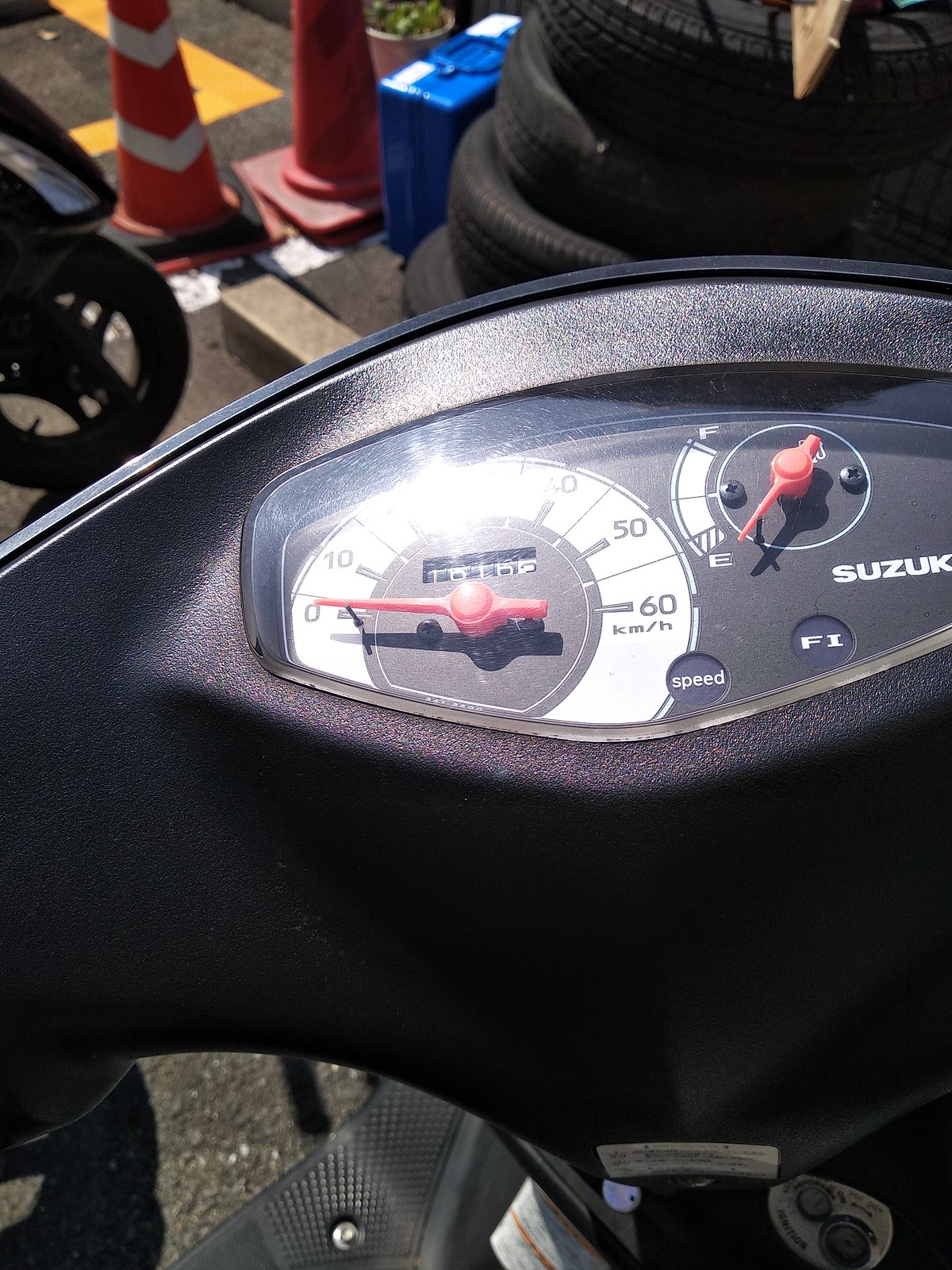The photograph captures an outdoor scene from the perspective of a motorbike rider seated on a Suzuki motorcycle. The view focuses on the handlebar area, prominently showcasing the brand name "SUZUKI" printed in white capital letters on the driver display. The display is encased in a black vinyl cover surrounding an oblong-shaped clear plastic cover, which shelters both the speedometer and gas gauge.

The speedometer, bordered by a white circle, marks speeds from zero to sixty kilometers per hour, with a red needle firmly pointing to zero, indicating that the motorbike is stationary. The plastic cover over the speedometer reflects bright daylight, especially around the twenty to twenty-five kilometer per hour marks. The adjacent gas gauge also features a red needle, currently pointing to empty.

In the foreground, just beyond the motorbike's handlebars, three rubber tires are stacked on the ground. Further into the distance, at the top of the image, a couple of orange traffic cones are visible. Additionally, the front tire of another motorbike can be seen in the upper left corner, hinting at a setting that involves multiple motorcycles.